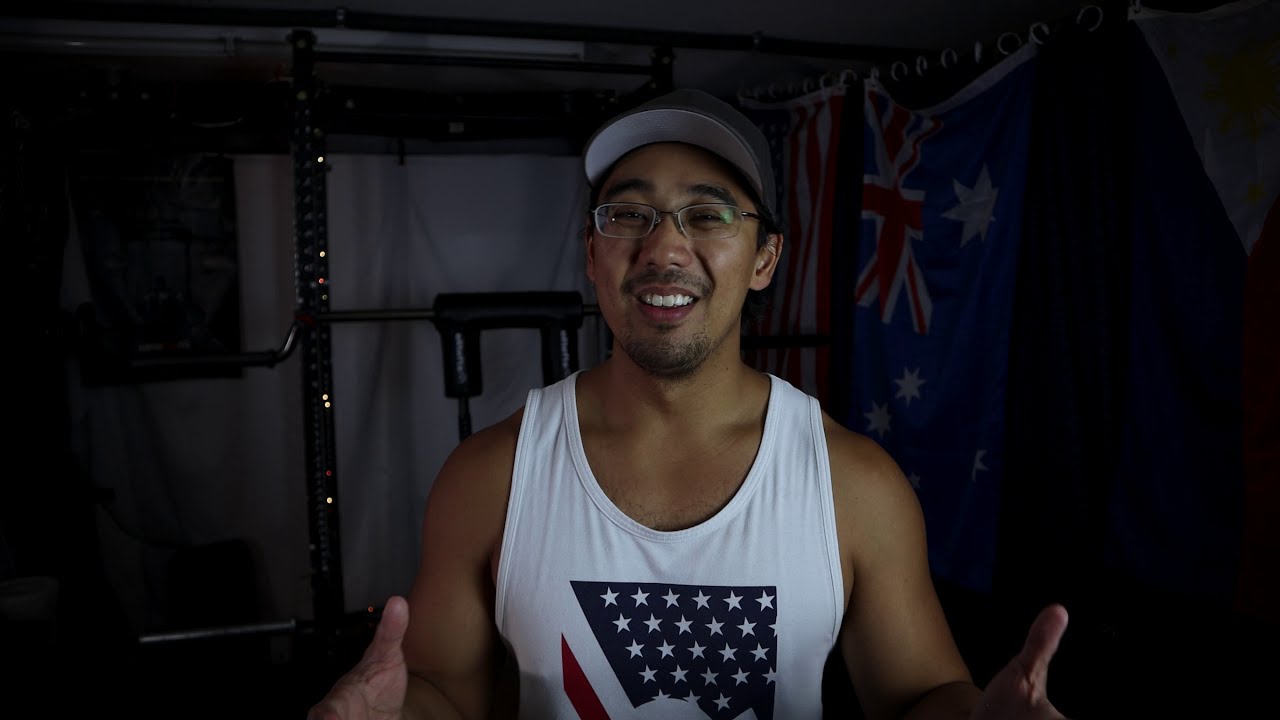In the center of the image stands a man of possible Asian descent with tan skin, wearing a baseball cap and glasses. He has a mustache and a beard along his jawline. He's dressed in a white sleeveless t-shirt that features a pattern reminiscent of the American flag, showcasing blue with white stars, complemented by red and white straps. The man appears to be mid-conversation, visibly smiling with his upper teeth showing, and has both arms extended as if he's explaining something enthusiastically. 

Behind him, there is equipment that resembles a home gym setup, including a barbell rack suitable for squats. The backdrop includes various elements: a black shelf holding some poles, an American flag with its distinct stars, and another flag that resembles a British flag with a red cross. The background seems adorned with different fabrics, from white sheets to flag patterns. The overall palette of the image includes red, white, blue, black, white, gray, silver, and some shades of brown, pink, and tan. The setting and his animated expression suggest the image might be a still taken from a vlog related to weightlifting or fitness.